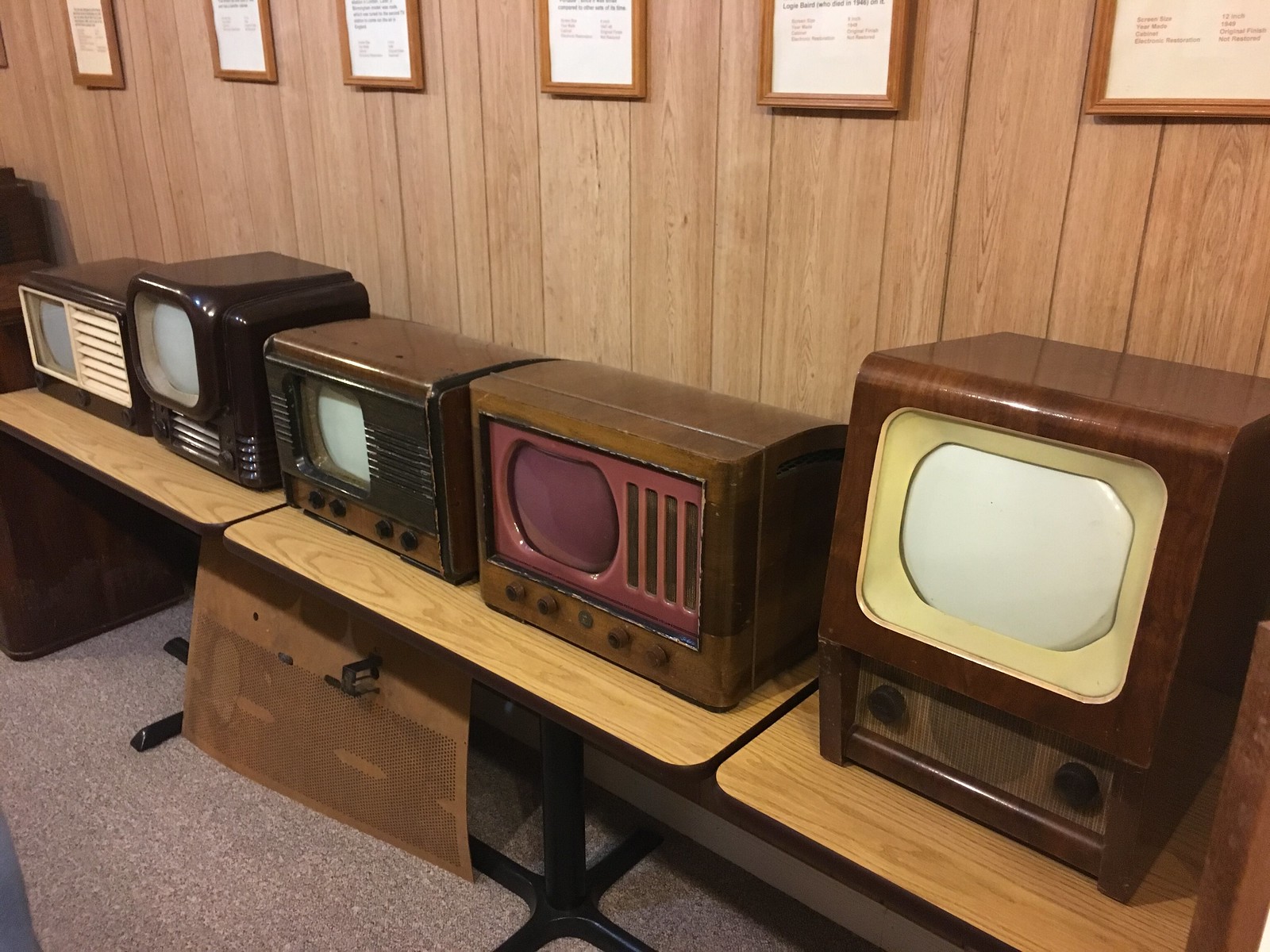This detailed color photograph captures a nostalgic scene featuring five small antique televisions positioned on a series of brown wooden tables. Each TV, ranging in size and design, showcases its vintage charm, with most having brown dials and some varying color accents around the screens. The TVs are angled slightly, moving from the bottom right to the top left of the image, enhancing the sense of depth.

The background is a light brown wood-paneled wall, complementing the wooden tables below. On the wall above the televisions are several small picture frames containing text in black and red on a white background, likely providing descriptions about each TV. These are encased in brown wooden frames that match the aesthetic of the wall and furniture. The carpeted floor features a reddish-brown and white pattern, adding a touch of color to the overall brown-toned room. In the left corner of the photograph, there is a noticeable blue object, adding a pop of contrasting color to the warm palette.